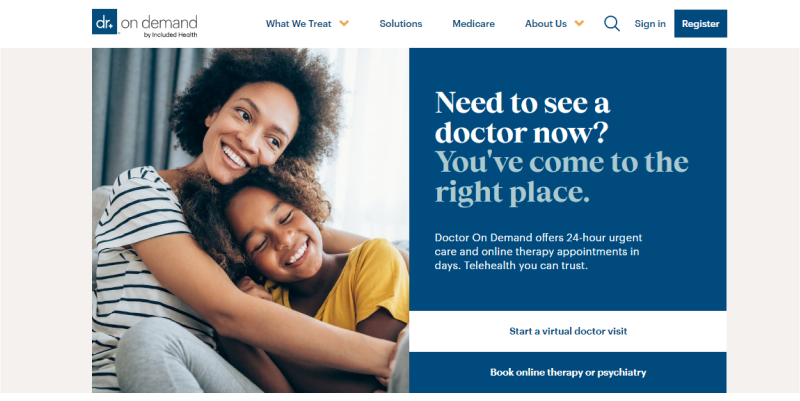The image portrays a web page for "Doctor on Demand by Included Health." At the top of the page, there is a navigation bar that includes several elements: a blue square with the word "Doctor" and text "On Demand by Included Health" beside it. The menu also has options such as "What We Treat" with a dropdown arrow, "Solutions," "Medicare," "About Us" with another dropdown arrow, a magnifying glass icon for search, and vibrant blue buttons for "Sign In" and "Register."

The central advertisement features a striking black woman with short curly hair, dressed in a white and blue striped shirt, seated in front of gray curtains while embracing a charming little girl. The young girl has similarly curly hair that reaches her ears, is dressed in a bright yellow blouse, and is smiling with her eyes closed, showcasing her beautiful white teeth.

Adjacent to their picture, a text box reads, "Need to see a doctor now? You've come to the right place. Doctor on Demand offers 24-hour urgent care and online therapy appointments in days. Telehealth you can trust." Below this statement, a white band with blue text prompts users to "Start a virtual doctor visit," and a blue box beneath it encourages users to "Book online therapy or psychiatry." This advertisement is for the telehealth service "Doctor on Demand" by Included Health.